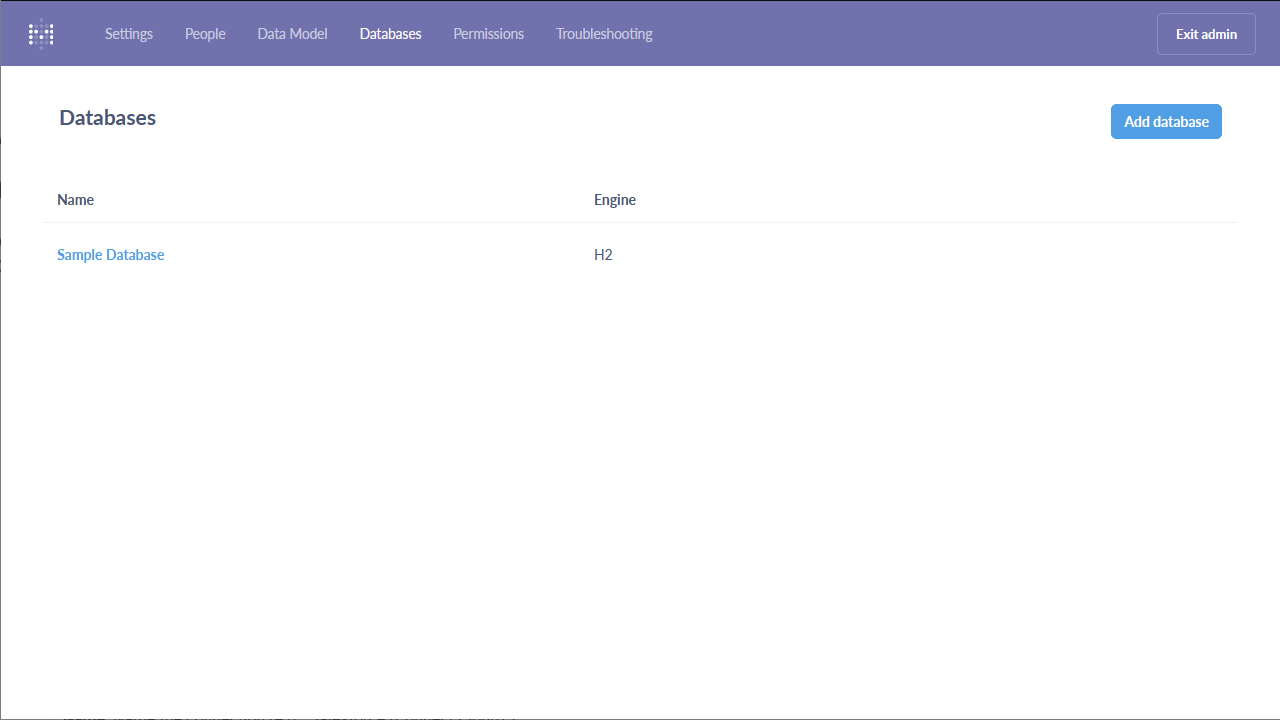The image is a screenshot with a clean white background, bordered by a thin black rectangle. Across the top of the screen, there is a lavender-blue bar stretching horizontally. On the far-left side of this bar is an icon resembling a capital "M" constructed from a series of small white circles. Adjacent to this icon is a series of labels in white text: "Setting," "People," "Data Model," "Databases," "Permissions," and "Troubleshooting." 

On the far-right end of the lavender-blue bar, there is a white rectangle containing white text that reads "Exit Admin." The currently active tab is the "Databases" tab, which is highlighted below the lavender-blue bar. Underneath this bar, the content area has a white background with the title "Databases" written in black text. 

On the extreme right side of the screen, near the top, there is a prominent blue rectangle button with white text that says "Add Database." Below this button, the section displays a heading in blue text "Name," followed by a subheading in black text "Sample Database," and another heading "Engine," with the value "H2" displayed in blue text.